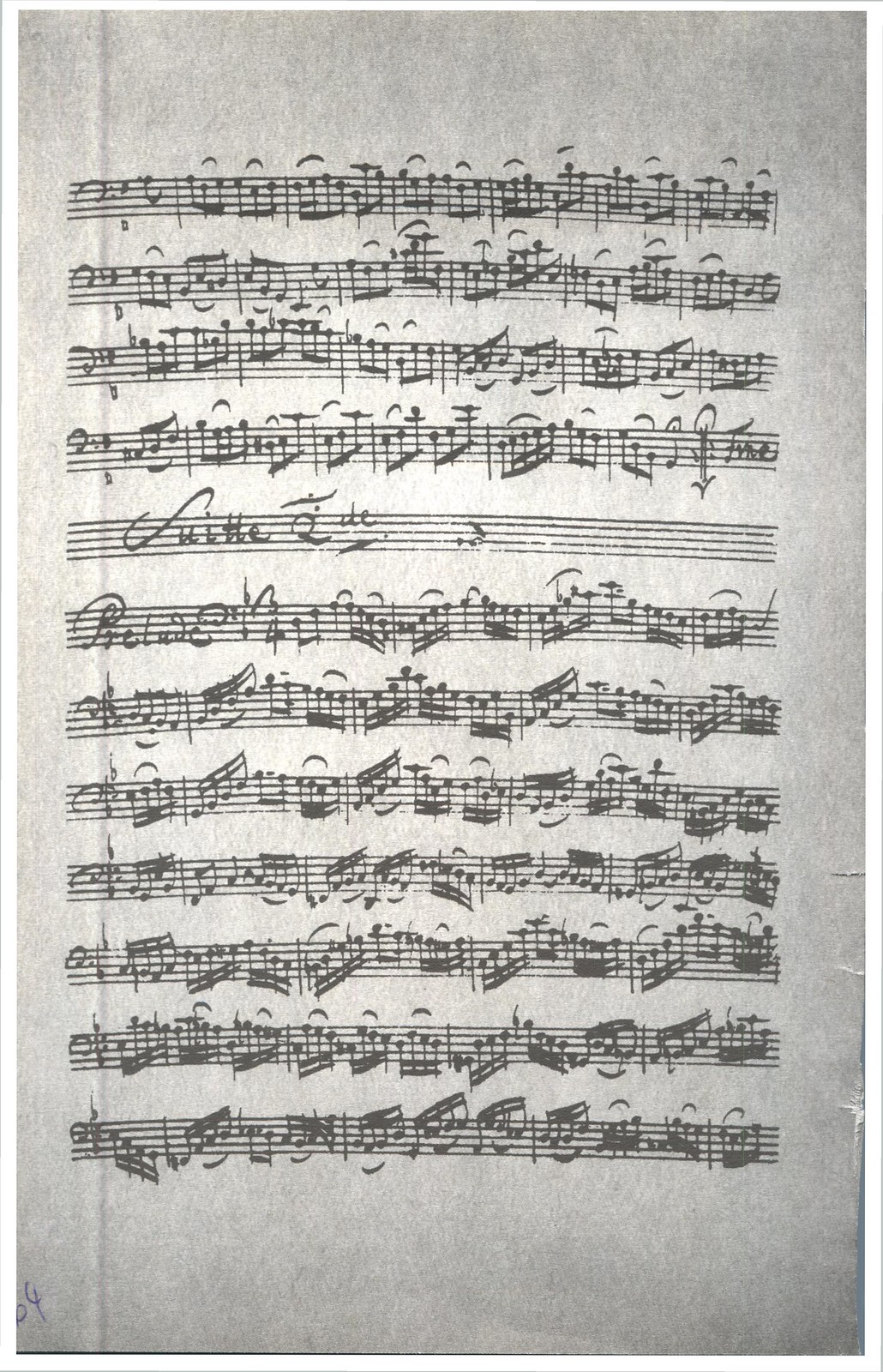The image showcases a black-and-white scan of a piece of sheet music. The sheet is predominantly white, serving as the background for twelve horizontal lines of musical notation, which occupy approximately three-fourths of the image, centered vertically with white margins above and below. Each of these twelve lines is densely populated with a variety of musical notes, suggesting a complex and possibly fast-paced composition. On closer inspection, the bottom left corner of the sheet reveals numbers inked in, likely "6" and "4." However, some wear and imperfections are visible, such as rips along the right side near the quarter mark of the page, indicating the paper's age or frequent use. Despite its intricacy and rich musical detail, the exact purpose—whether for practice or performance—remains ambiguous.